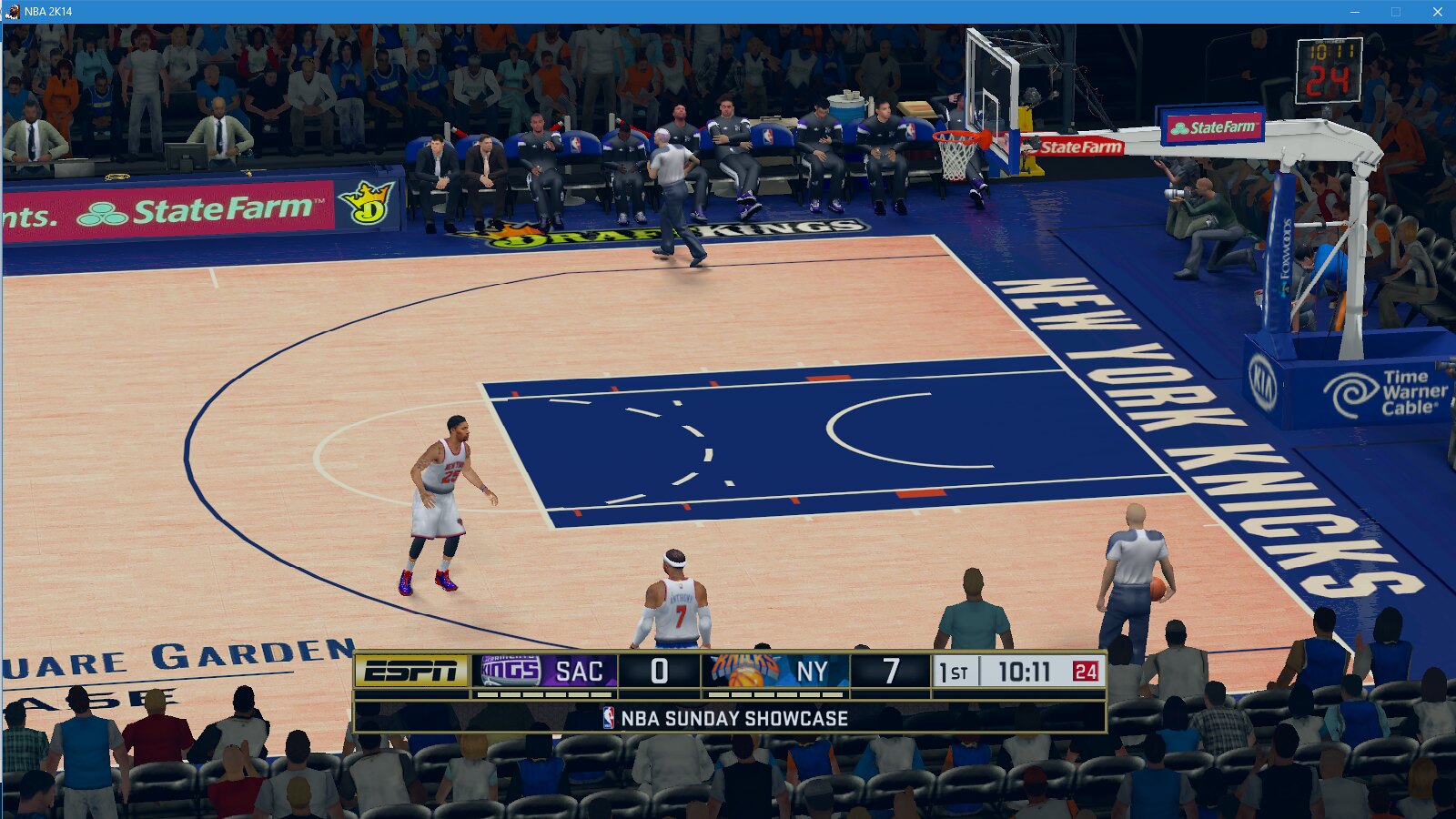This image is a highly realistic still from an NBA-themed video game, capturing the intensity of an NBA Sunday Showcase between the New York Knicks and the Sacramento Kings. At the bottom of the image, a row of spectators occupies folding chairs, providing a vibrant backdrop. The court, featuring a wooden floor with a navy blue painted key area, prominently displays "New York Knicks" and "Square Garden," indicating the iconic Madison Square Garden. A basketball hoop extends over the blue key, and the semi-circle three-point line is visible. On the court, Knicks player number 7 stands ready, while a referee, with a ball under his arm, positions himself at the bottom right.

The scoreboard shows a score of 7-0 in favor of the New York Knicks against Sacramento, with the banner displaying "NBA Sunday Showcase" and sponsors including ESPN and State Farm. Additional advertisements for Time Warner Cable and Draft Kings encircle the court. The rich detail includes fans around the perimeter, broadcasters, and a lively game atmosphere, making the scene highly immersive.